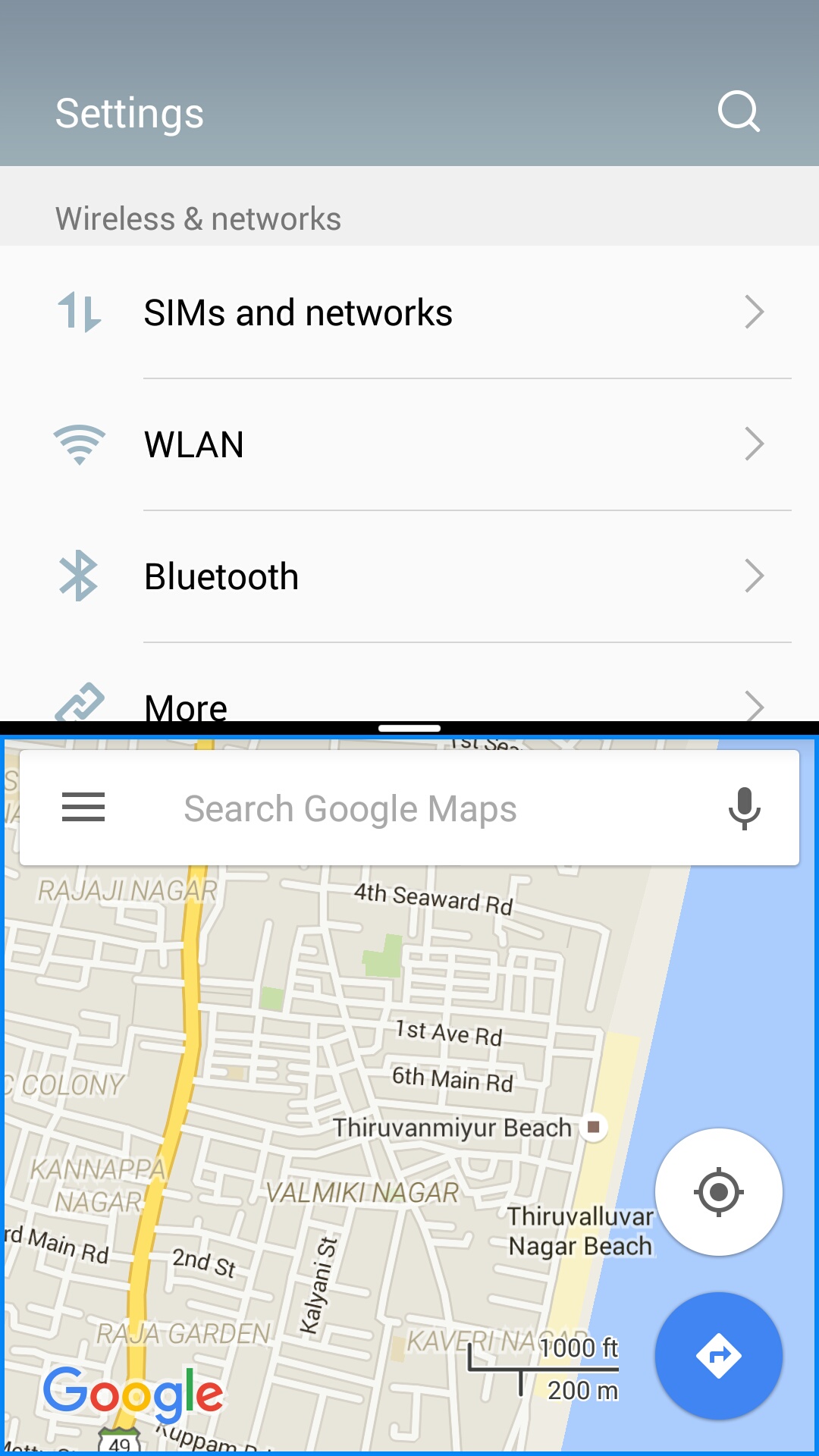This image, displayed on a phone screen, shows the settings menu with a distinctive layout and sections. At the top, there's a gray bar containing a search icon. Below this, a light gray section is labeled "Wireless and Networks." Further down, an even lighter gray section lists various options including "SIMs and Networks," "WLAN," "Bluetooth," and "More."

Continuing down the screen, there's a section featuring a Google Maps interface. This includes a search bar labeled "Search Google Maps," accompanied by a microphone icon on the right side. On the left-hand side, there are three horizontal bars indicating the menu options.

The map itself is mainly beige, with the primary road highlighted in yellow, labeled "Rajanagar." The map also features "Thiruvivarnagar Beach," suggesting the location could be in a different country. 

In the bottom left corner, the Google logo is present, characterized by its iconic colors: blue, red, yellow, blue again, green, and red. On the right side of the map, light blue shading indicates a body of water.

Additionally, there are two notable circular icons on the right side: one blue circle with a white diamond in the middle, and another white circle with a black and white image that has a central circle.